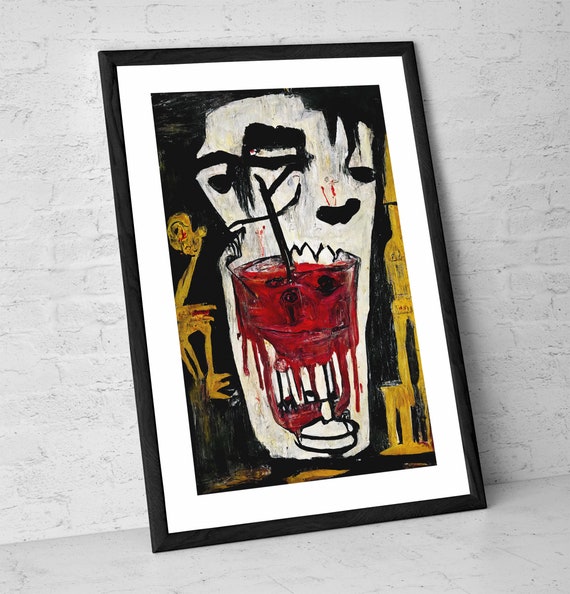This is a photograph of an abstract painting, framed in glass with a white mat and black trim, leaning against a white brick wall with a tiled floor. The central focus of the painting features a glass filled with red liquid, potentially resembling blood or Kool-Aid, with a black straw protruding from it and red liquid seeping from the bottom. Behind the glass, there appears to be a ghost-like figure with white and gray shading and black markings. To the left of this figure, there's an image of a humanoid with a yellow-orange face displaying facial features such as an eye and eyebrow, with peculiar red-streaked arms extending from it. On the right-hand side, there's a church-like building in a green, lime hue with a high steeple, and nearby, an ambiguous golden object. The painting also contains two intertwined, white ghostly faces, one more prominent than the other, and dark, eerie skeletal limbs disjointedly arranged through the composition.